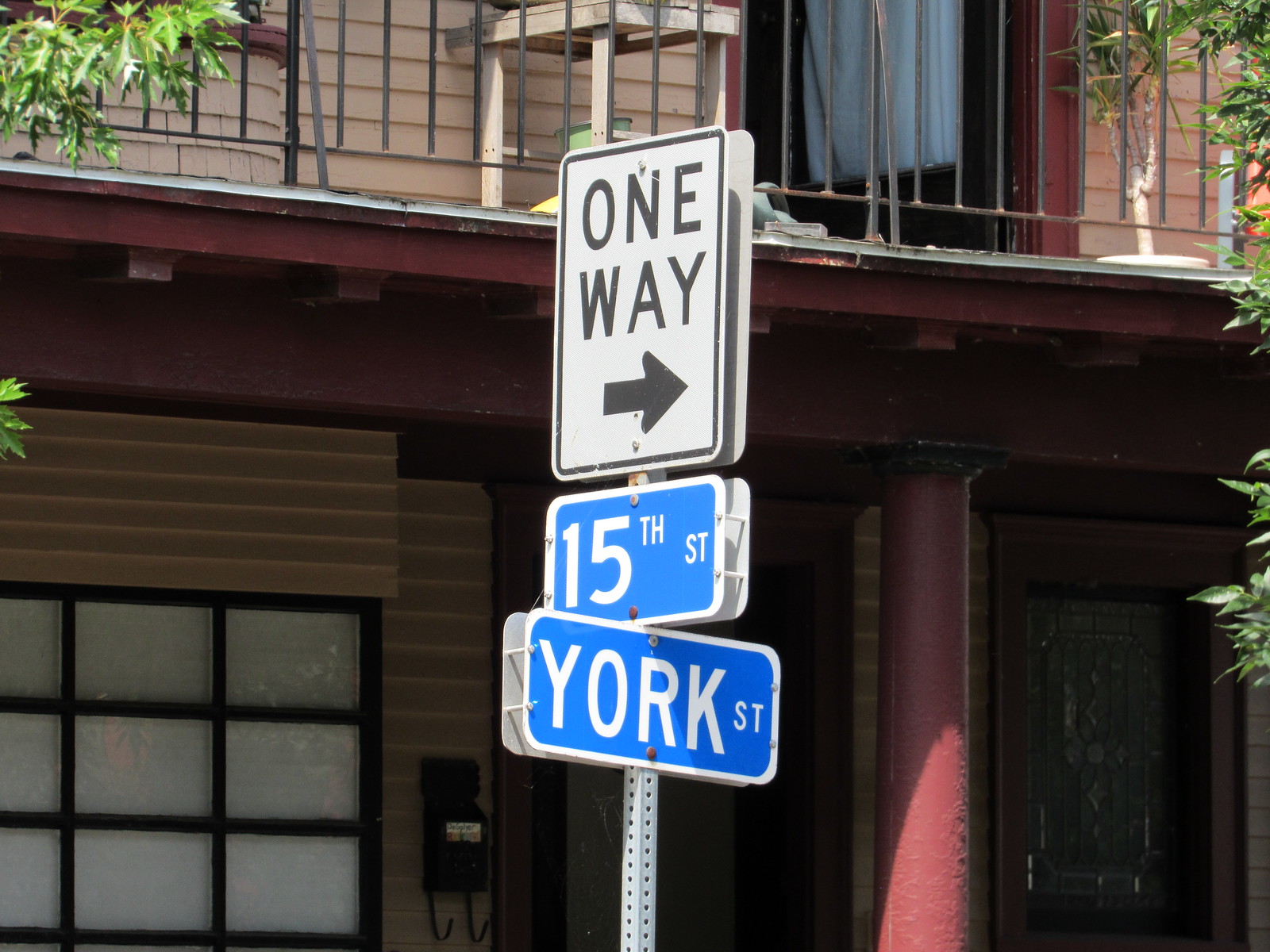The image captures a well-lit, sunny scene of a residential intersection featuring a prominent street sign. At the top of the steel pole, a white "One Way" sign with black lettering and a right-pointing arrow is clearly visible. Below it, two blue street signs with white letters indicate "15th Street" and "York Street," positioned one beneath the other. Set against the backdrop is a two-story building that appears to be an apartment or condominium, characterized by different hues of maroon siding on the upper level, a maroon-trimmed lower level, and a maroon pillar. Notable details include a black-framed window, a black mailbox with an open top attached near a front door featuring a stained glass design, and a white table on an upper-level balcony, which is framed by a railing. The surroundings are enhanced by the presence of green trees and leaves at the edges of the photo, adding a vibrant touch to the residential setting.